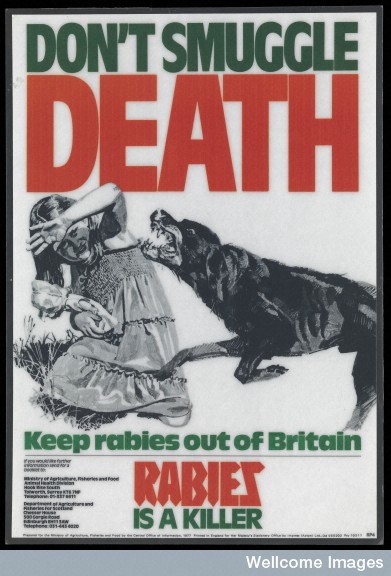The image shows an old-fashioned, anti-rabies poster with a black and white illustration. At the top, in bold green text, are the words "Don't smuggle" followed by the word "death" in very large red letters. "Don't smuggle death" is prominently stated. Below this text, there is a black and white picture of a little blonde girl in a sundress. She is sitting on a tuft of grass, clutching a doll and shielding her eyes with her arm. A rabid-looking dog, possibly a Rottweiler, is lunging towards her with its teeth bared, appearing poised to attack. Below the image, the text reads "Keep rabies out of Britain" in green letters, underlined. Further down, in large red letters, it says "Rabies," followed by "is a killer" in green letters. The entire poster has a thin black border with an inner thin gray line. Additionally, there is some small, unreadable text in the bottom left corner of the image, and the name "Welcome Images" is noted in the bottom right corner, outside the poster's border.